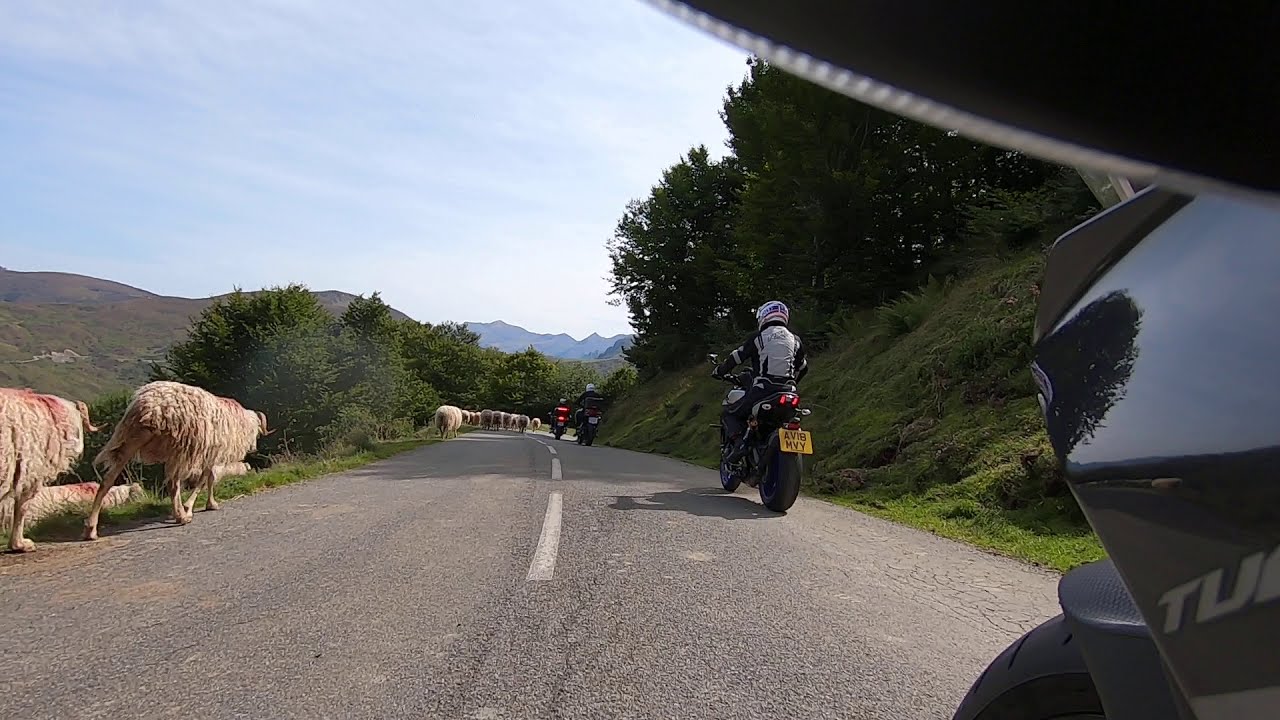The horizontally aligned rectangular picture captures a scenic mountain road flanked by lush greenery. The right side of the image features a grassy hillside peppered with rocks and topped with trees. In the foreground on the right, we observe the edge of a motorcycle, including part of its wheel, the black siding, and the letters "TU." A motorcyclist wearing a gray helmet, gray and black top, and black pants is visible further up the middle of the picture, traveling on a paved road divided by a white dotted line. Additional motorcyclists can be seen in the distance, also occupying the right lane.

On the left side of the road, a series of thick-wooled, horned creatures, possibly bulls or shaggy sheep, walk along the left lane, heading in the same direction as the motorcycles. The animals have beige fur and appear somewhat fuzzy. The background displays a clear blue sky with feathery white clouds, particularly noticeable in the middle and upper left portions of the frame. This detailed setting imbues the scene with a sense of adventure and an interplay between nature and human activity.